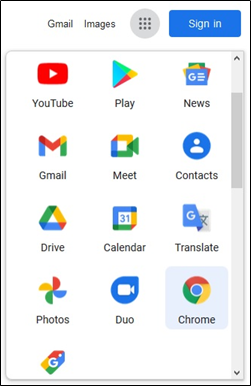The image depicts a screenshot of a Google services menu. At the top, the screen displays the text "Gmail" and "Images." Below, there is a gray circle icon with nine dots arranged in three rows, adjacent to a blue "Sign In" button. The menu lists various Google services, starting with YouTube, indicated by its iconic red play button, followed by Gmail with its recognizable envelope logo. Next is Google Drive, represented by a triangular icon in Google’s signature colors, and Google Photos. Additionally, there's an icon resembling a gift tag, also adorned with the Google logo.

Further up on the menu, prominent Google services such as Play, Meet, Calendar, and Duo are highlighted in blue. Lower down, the list includes News, Contacts (marked by a blue circle), Translate, and Google Chrome. On the right side of the screen, an up and down arrow indicates the availability of more content to scroll through. The screenshot features a white background with a thin black border, illustrating a user interface summarizing Google's diverse service offerings.